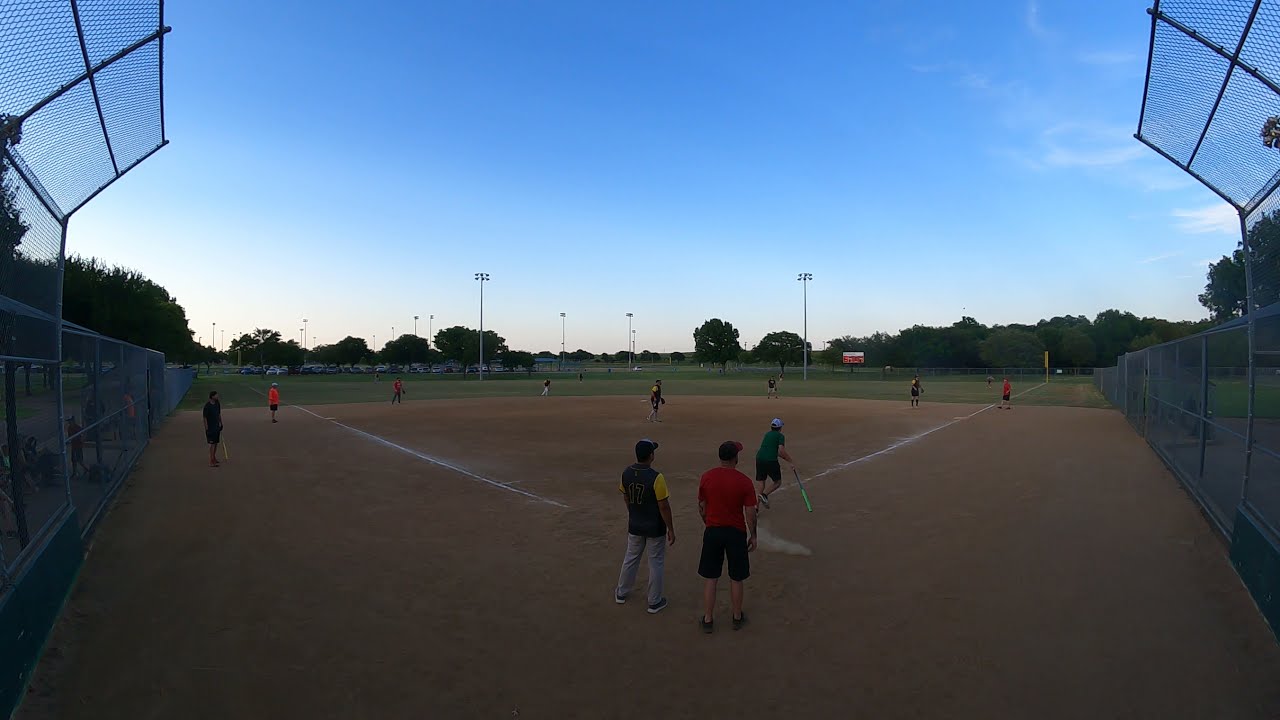The photograph captures a wide, rectangular image of a baseball diamond from a slight elevation behind the batter, near first base. The reddish-brown sand of the diamond dominates the bottom half of the frame, bordered with white paint, while the green grass of the outfield stretches beyond. At the edge of the field, a metallic net fence marks the boundary, curving at the top to the right. In the background, very tall gray stadium lights stand guard, casting their gaze over a parking lot filled with cars, and thick green trees line the horizon. The sky above is a light blue with only faint, transparent clouds in the top right corner.

In the center of the image, two men stand watching the game. The man on the right, wearing a red shirt, black shorts, and a ball cap, is accompanied by a man to his left, dressed in jeans, a blue shirt, and also a ball cap. On the field, a batter in a green t-shirt and black shorts appears to have just hit the ball and is running toward first base, still holding the bat. Other casually dressed players are visible, positioned at various bases and out in the green outfield. To the left of the two men, another pair of men stand by the fence, augmenting the scene of engaged spectators and players. Toward the right of the parked cars, a scoreboard is visible, and to the far right, the trees create a natural border, completing the vibrant and detailed panorama of the baseball game.